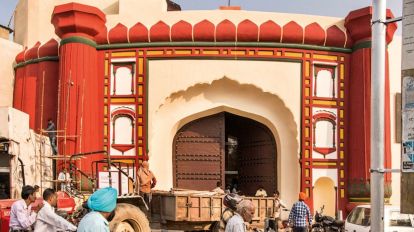This photograph captures the vibrant exterior of a heritage building that boasts an architectural style reminiscent of an Indian castle or Mughal-era monument. The structure is intricately painted in a palette of red, cream, and yellow. Dominating its facade are two giant red pillars flanking a wide, castle-like, arched wooden entrance door with grooved floral designs, exuding historical charm.

The building's cream-colored walls and roof are complemented by red and yellow inlaid paintings, with rectangular trims and rounded curved red framing. A faintly visible flag on top hints at its cultural significance. In front of the building, the scene is bustling with activity: people wearing blue and orange turbans and others driving motorbikes and tractors traverse the sunlit road. A metallic white pole and various signboards dot the area, providing context to the lively street environment under a clear blue sky.